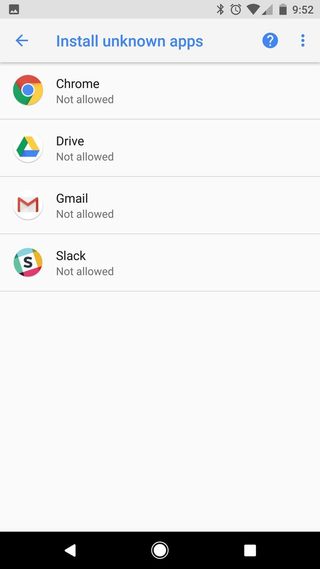The image displays a screenshot from the "Settings" app of an Android phone, focusing specifically on the "Install Unknown Apps" section. At the top of the screen, bold blue text reads "Install Unknown Apps," accompanied by a left-pointing arrow and a blue question mark icon, which appear to be elements for navigation and help, respectively.

Below the title are several app entries, each accompanied by their respective icons and "Not allowed" status:
1. **Chrome** - Represented by the traditional red, green, yellow, and blue circular logo.
2. **Drive** - Presumably Google Drive, denoted by its classic green, yellow, and blue triangular logo.
3. **Gmail** - Identified by the white envelope with a red "M" overlay.
4. **Slack** - Marked by an "S" with a distinctive checkerboard, multi-colored pattern.

At the bottom of the screen is a black navigation bar featuring a home button, a back button, and a square-shaped button, typical of many Android interfaces.

The status bar at the top indicates several details: the current time displayed as 9:52, a nearly full battery icon, symbols for an alarm and Bluetooth, and additional, less discernible icons. The overall background of the screen is a traditional grayish tone, characteristic of many default Android settings screens.